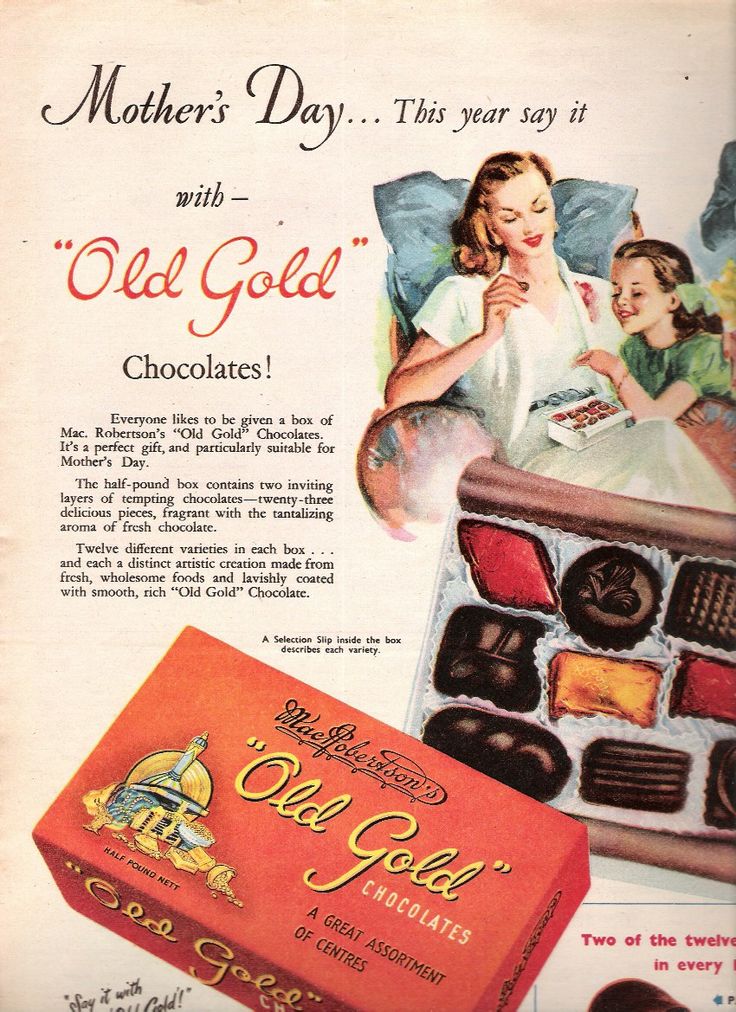This vintage magazine advertisement for Mac Robertson's Old Gold Chocolates, likely from the late 1940s or early 1950s, is targeted for Mother's Day. The ad features a large heading at the top, stating: "Mother's Day this year, say it with Old Gold Chocolates." The central image depicts a fair-skinned woman in a white gown, seated in an armchair, with her blonde-haired daughter in a green dress and green hair ribbon by her side. They are both admiring a box of chocolates with evident delight.

The advertisement also shows an opened red box of Old Gold Chocolates, displaying an assortment of differently shaped chocolates. The box at the bottom includes vividly wrapped chocolates in red and gold, indicating a luxurious presentation. The tagline emphasizes the universal appeal: "Everyone likes to be given a box of Mac Robertson's Old Gold Chocolates. It's a perfect gift and particularly suitable for Mother's Day."

Detailed descriptions underscore the product's allure: "The half-pound box contains two inviting layers of tempting chocolates, 23 delicious pieces fragrant with the tantalizing aroma of fresh chocolate. Each box features 12 different varieties, each a distinct artistic creation made from fresh, wholesome foods and lavishly coated with smooth rich Old Gold Chocolate." Additionally, a selection slip inside the box describes each variety in detail.

The ad, tinged with a sepia tone indicating its age, also features an illustration of a palace and scattered gold accents, reinforcing the idea of opulence associated with these chocolates. The overall composition, in full color, vividly evokes a sense of nostalgia and classic elegance.